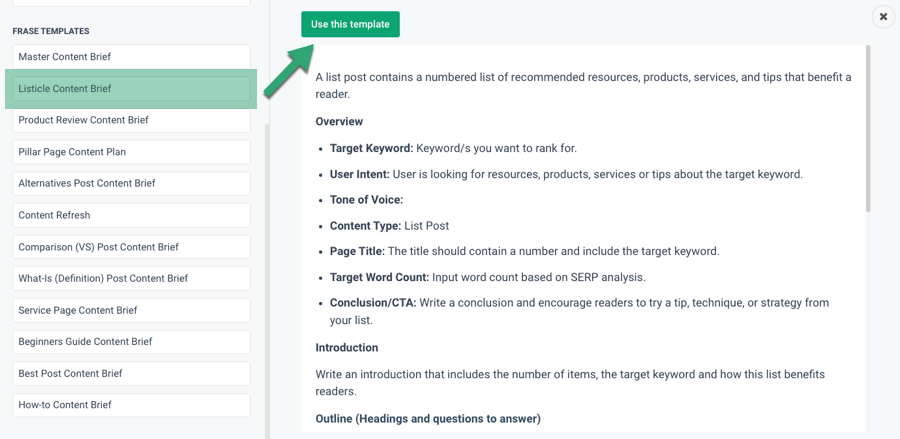This image displays a section of a web page focused on "Phrase Templates." The top-left corner features the header "Phrase Templates" in bold black text on a gray background. Above this section, there is a partially visible white area, indicating another section of the page that is cut off.

Beneath the header, various rectangle boxes offer different selections. The second selection is highlighted in light green, with a slightly darker green arrow pointing to a button labeled "Use This Template." This template is described as a "list post" designed to provide a numbered list of recommended resources, products, services, and tips beneficial to readers.

The main body of the page includes an "Overview" section, followed by a bulleted list that outlines key elements such as:
- Target word
- User intent
- Tone
- Voice
- Content type
- Page title
- Target word count
- Conclusion/CTA (Call to Action)

An introduction is specified, instructing the user to write an introduction that includes the number of items, the target keyword, and how the list benefits readers. Below the introduction, there is an "Outline with information" section in parentheses.